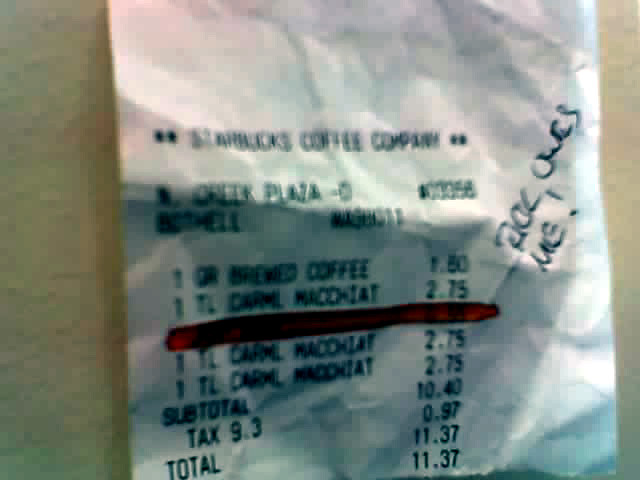The image features a crumpled receipt laid out on a white tabletop. The receipt is printed on standard white receipt paper and shows the header "Starbucks Coffee Company, O'Reilly Plaza," followed by some partially legible text. The list of ordered items includes a brewed coffee, three caramel macchiatos, and a fourth item that is highlighted in red but obscured and unreadable. Handwritten in pen, the note "Rick owes me" is visible on the receipt. The subtotal for the items is $10.40, with a calculated tax of 9.3% amounting to $0.97, bringing the total to $11.37.